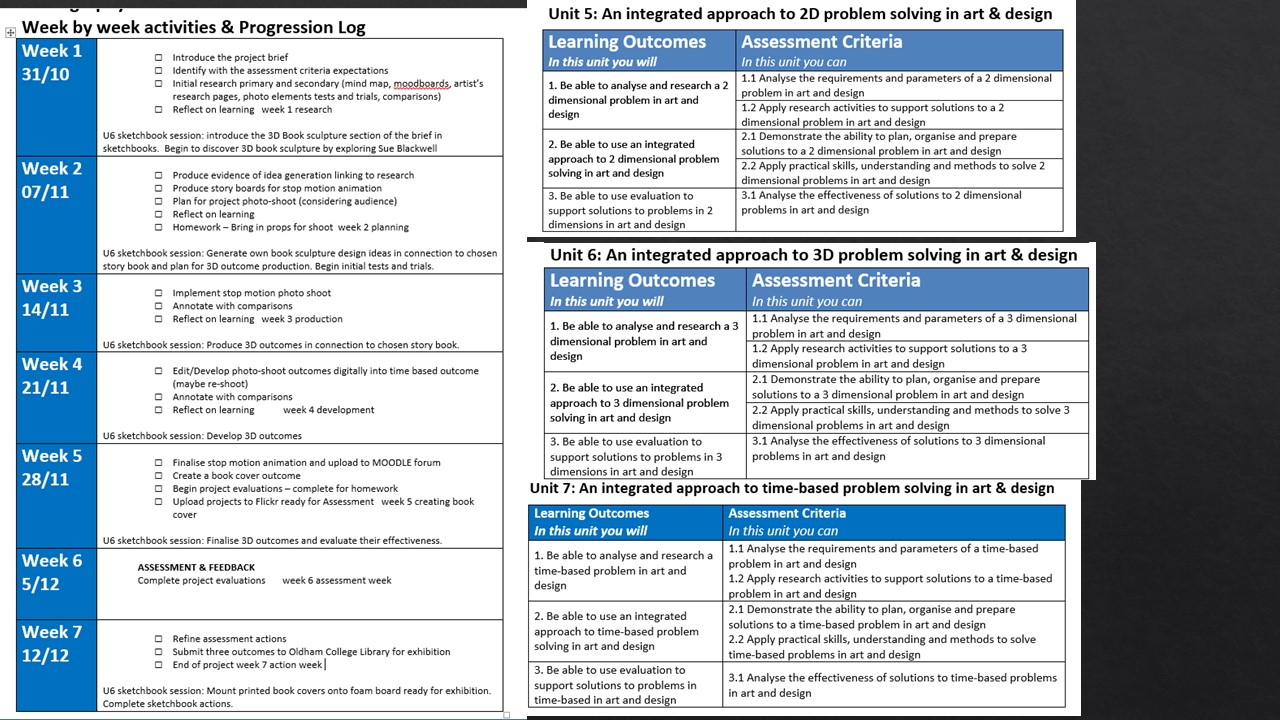The image is a detailed curriculum visually formatted with a week-by-week activities and progression log, primarily for Unit 5, which emphasizes an integrated approach to 2D problem solving in art and design. It starts with week 1, dated 1-10, where the project brief is introduced, assessment criteria expectations are identified, and initial research begins, including primary and secondary data collection, mind mapping, creation of mood boards, and artist research pages. It also involves photo elements, trials, comparisons, and reflections on the research conducted. In week 2, dated 7-11, the focus shifts to generating ideas linked to the research, producing storyboards for stop motion animation, planning for a project photo shoot with audience consideration, and reflecting on the learning process. Additionally, there is a homework task to bring in props for the shoot. The right side of the image outlines learning outcomes and assessment criteria for Unit 5, along with Unit 6, which deals with 3D problem solving, and Unit 7, which focuses on time-based problem solving in art and design. The schedule is presented on a white background with distinctive blue blocks denoting dates and weeks, featuring black font text for detailed instructions.